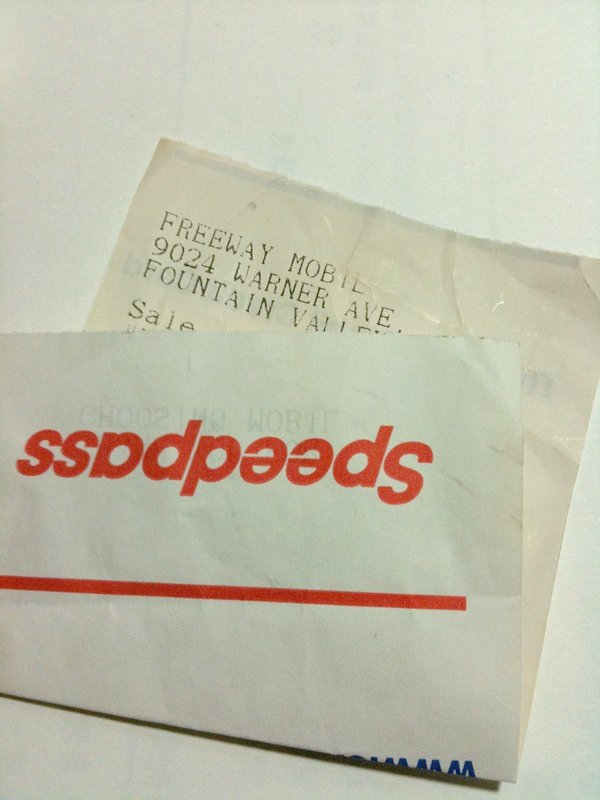A photograph captures a folded receipt resting on a clean, white surface. Prominently displayed in red text on the receipt is the phrase "Speed Pass." At the top in black font, the text reads "Freeway Mobile," followed by an address, "9024 Warner Avenue," but the name of the town, presumably "Fountain Valley," is partly obscured due to the folding. The word "Sale" is also visible. The remainder of the receipt's details are hidden by the folds. On the reverse side, near the Speed Pass text, a few letters in blue are visible, although they are not legible enough to determine what they say.